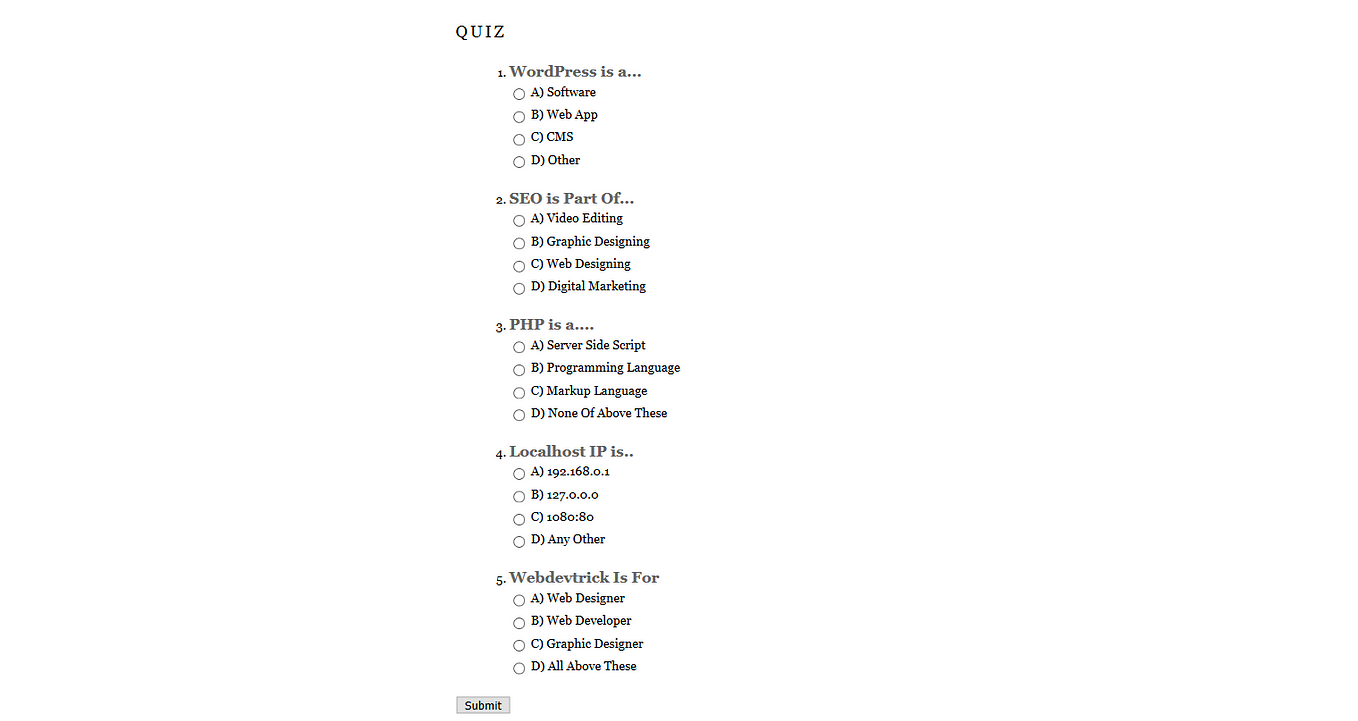Screenshot of an online quiz interface with "QUIZ" prominently displayed in the top left corner in uppercase letters. The quiz consists of four multiple-choice questions each followed by answer options labeled A, B, C, and D with radio buttons for selection:

1. **WordPress is a...**
   - A) Software
   - B) Web App
   - C) CMS
   - D) Other

2. **SEO is a part of...**
   - A) Video Editing
   - B) Graphic Designing
   - C) Web Designing
   - D) Digital Marketing

3. **PHP is a...**
   - A) Server-Side Script
   - B) Programming Language
   - C) Markup Language
   - D) None of the Above

4. **Localhost IP is...**
   - A) 192.168.0.1
   - B) 127.0.0.1
   - C) 10.0.0.1:80
   - D) Any Other